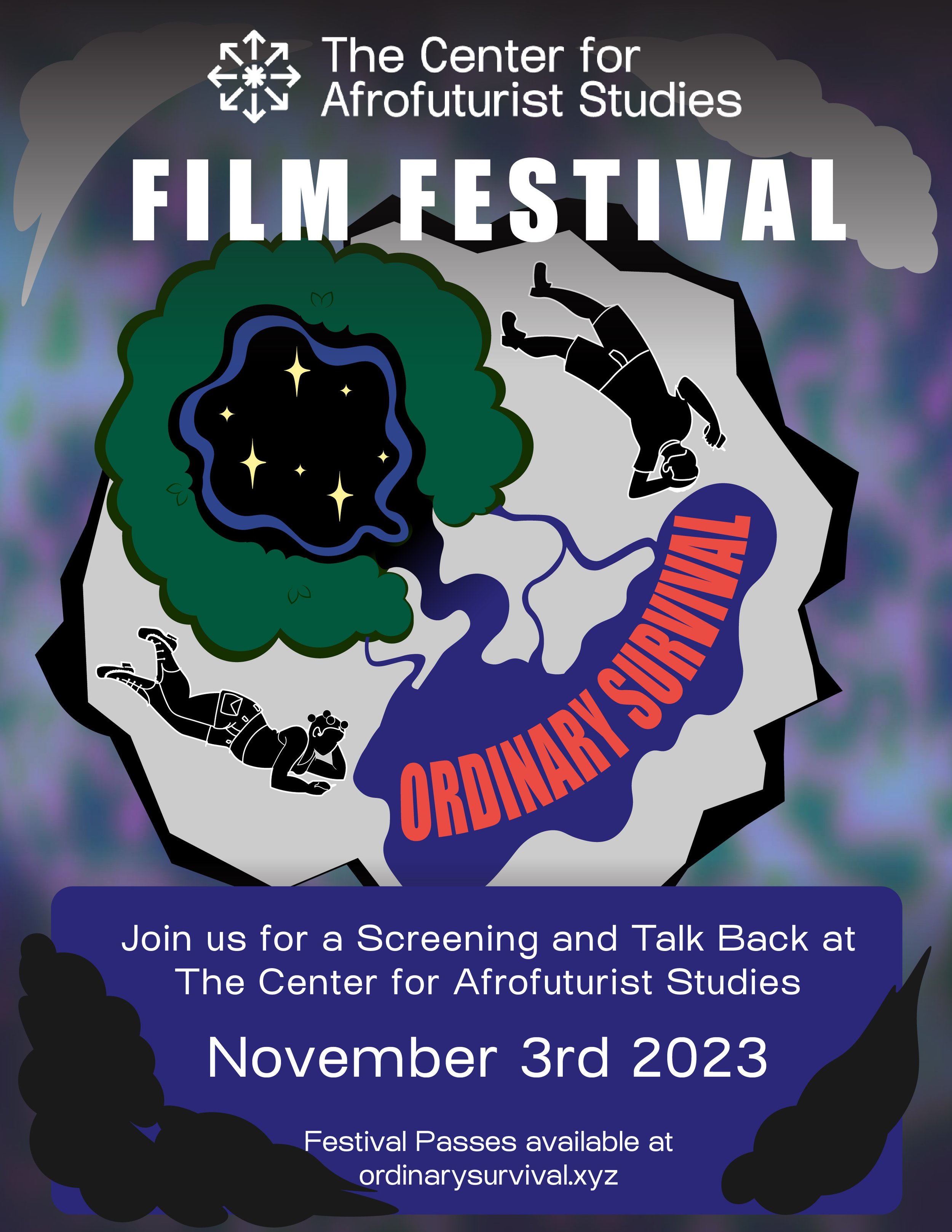The poster for the Center for Afrofuturist Studies Film Festival prominently features the title "Ordinary Survival" in bold red capital letters. At the top, the text in white letters announces "Center for Afrofuturist Studies" followed by "Film Festival." The central image has a cartoonish aesthetic depicting a man and a woman lying down on either side of a landscape featuring a lake and a starry sky. The scene is enclosed within a circular design with elements of trees and stars. The lower portion of the poster invites viewers to "Join us for a screening and talk back at the Center for Afrofuturist Studies, November 3rd, 2023." It provides further information that festival passes are available at OrdinarySurvival.xyz. The overall color scheme of the poster primarily includes blues and greens, contributing to its visually striking appearance.